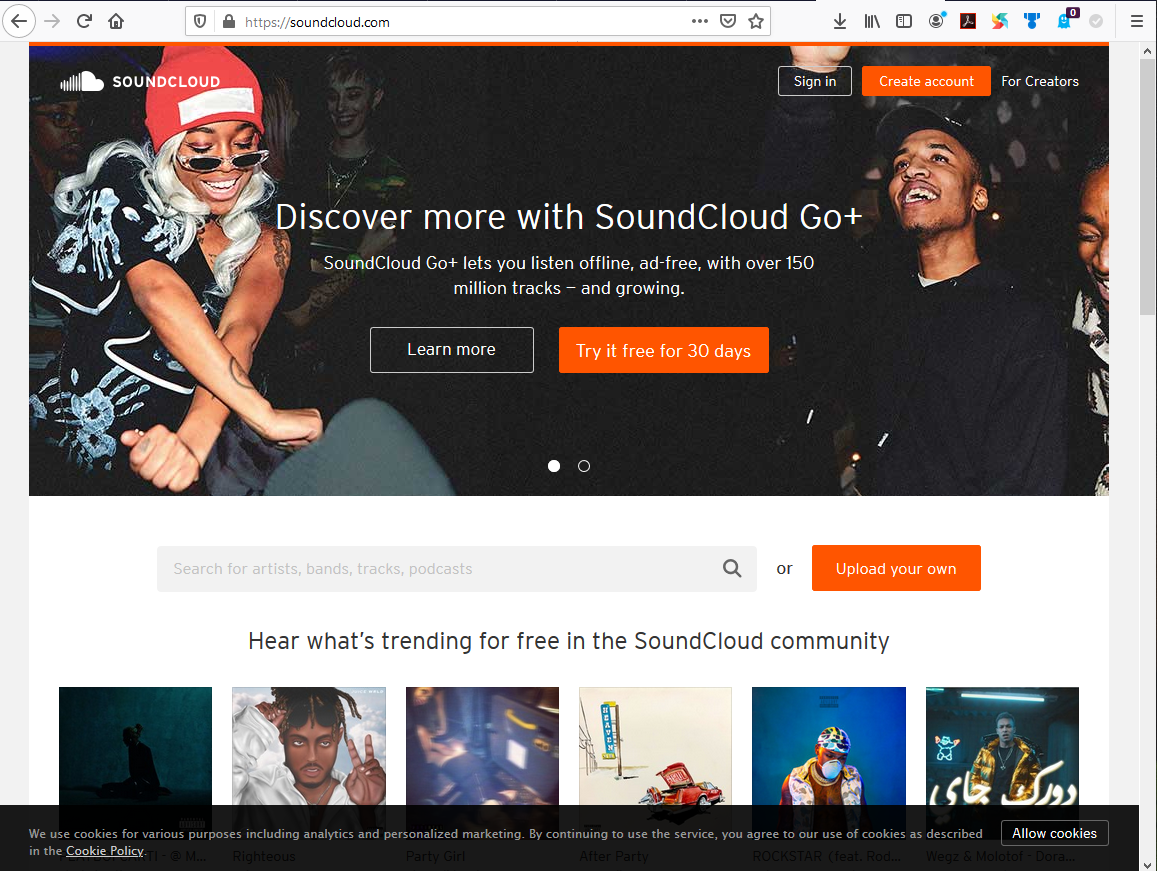The image depicts the homepage of SoundCloud's website. The screen is slightly dimmed, framing two individuals with dark skin tones in the background. The girl on the left is distinctive with her white hair and a red cap, which features a partially obscured label. The SoundCloud logo is prominently displayed in the upper left-hand corner, consisting of a stylized cloud that is half solid white and half striped white.

Key elements of the webpage are visible, including a search bar at the top where "SoundCloud" is written, allowing users to search for content. Users have the options to sign in or create an account, as indicated in the upper right-hand section. The site promotes its premium service, SoundCloud Go+, with a banner that highlights benefits such as offline listening, an ad-free experience, and access to over 150 million tracks. The promotional message is accentuated with buttons to "Learn more" in a black box and "Try it for free for 30 days" in a red box.

Further down, the webpage features sections for discovering and trending music within the SoundCloud community, showcasing six artist images that are partially obscured by a black banner with white text. This banner informs users about cookie usage, offering links to read the cookie policy or accept cookies.

The image appears to have been captured from a computer screen, as evidenced by the visible browser icons at the top and various menu icons along the left-hand side.